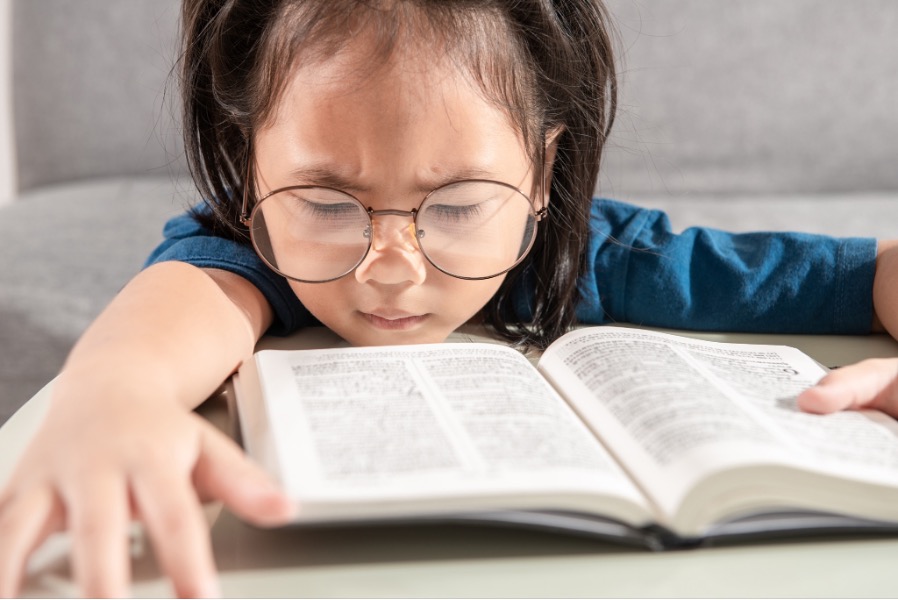In the image, a young child, appearing to be between five and nine years old, is engrossed in a book sprawled out on a low piece of furniture, like an ottoman or a coffee table. The child is kneeling between a gray couch and the low object, stretching their arms over it to read the open book, which contains very tiny words in a two-column layout, suggestive of a scriptural text such as a Bible or Koran. Wearing a blue shirt with sleeves partially kited up and large circular wire-framed glasses, the child has longer brown hair that frames a face focused intently on the pages, squinting as if they are having difficulty reading the small print. The cozy, home-like setting enhances the intimate scene of youthful determination or sleepy intrigue.